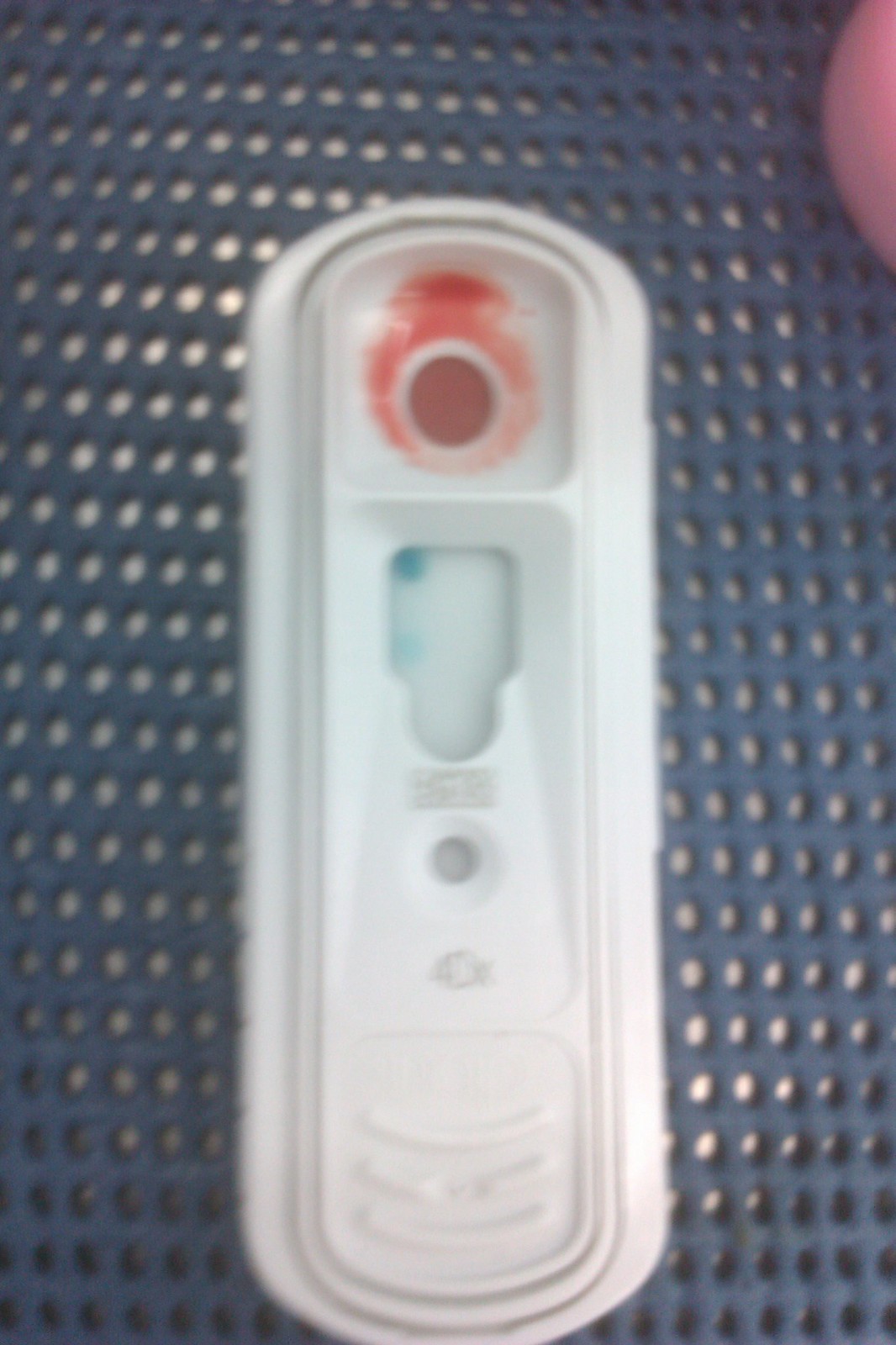This photograph features the inner components of a test device, potentially a COVID-19 or chlorine test kit. The background is a distinctive blue rubber mat, commonly found in swimming pool areas, characterized by multiple holes, which hints at potential use for water quality checks such as chlorine and alkaline testing. In the upper right corner of the image, there is a visible finger, suggesting human interaction with the test.

The test device itself is white and resembles a long, flat oval tablet. It contains two distinct wells. The first well, shaped like a piece of toast with a rounded top, has a central hole surrounded by a red-colored area. The second well is elongated and rectangular with rounded edges. This well features a keyhole-like shape marked by two blue spots on a predominantly white background. The detailed structural features and the colors within the wells suggest the different reagents or indicators used in the testing process.